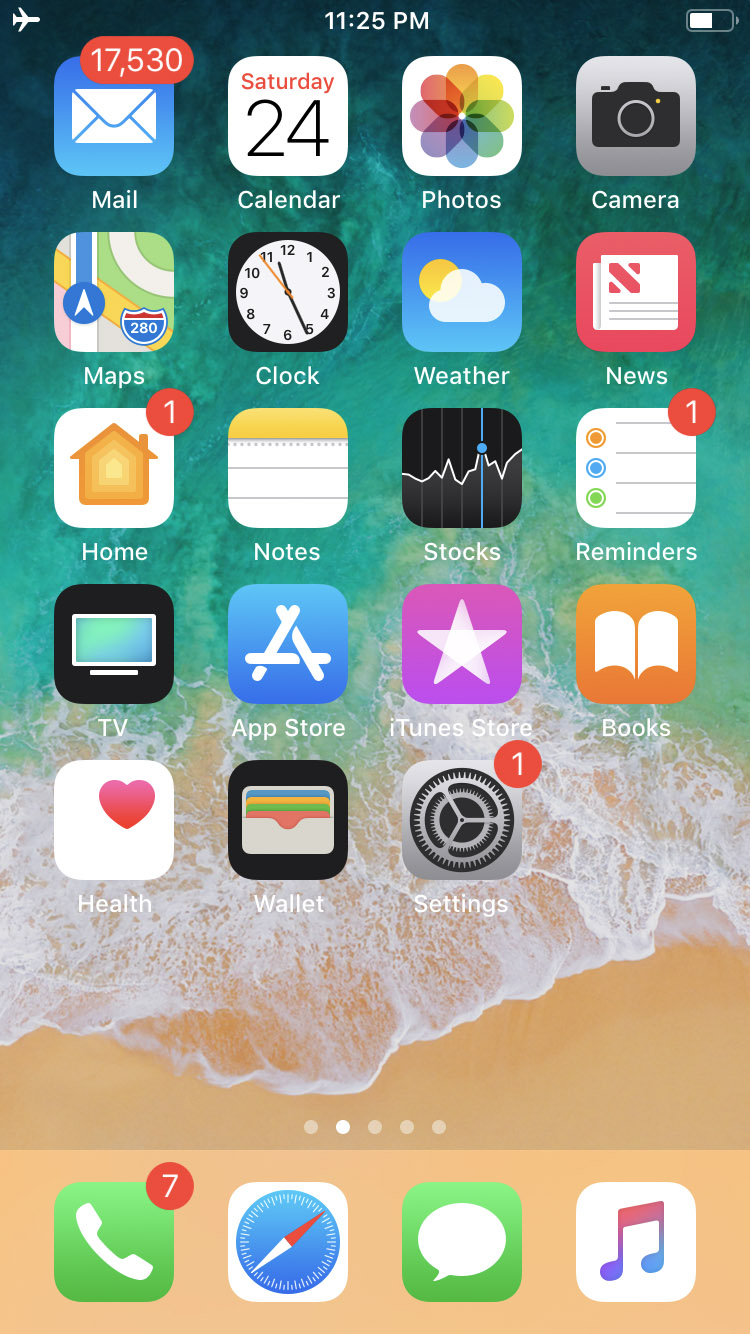A detailed screenshot from an Apple mobile device - presumably an iPhone or iPad - captured at 11:25 PM. The status bar at the top reveals crucial details: a white airplane icon indicating airplane mode at the upper left corner, the current time, and a half-full battery icon on the right. The background features an artistic, non-photorealistic wallpaper of a serene beach scene. The wallpaper transitions from dark bluish-green at the top to a vibrant green further down, with waves gently lapping at the sandy shore at the bottom.

The home screen is densely populated with various app icons. At the very top left, the mail icon in blue with a staggering 17,530 unread messages in red. Adjacent to it are the calendar, photos (depicted by overlapping colorful circles), and camera icons. The second row houses the maps, clock, and weather icons - the latter showing a sun peeking out from clouds on a blue background. This row also includes the news icon in red and white, the home app with a notification badge indicating one new item, the notes app, the stocks app, and the reminders app, which similarly displays one new reminder.

Further along, you'll find icons for the TV app (a black background displaying a TV screen), the App Store in blue, the iTunes Store with a white star on a pink background, the Books app, the Health app (with a white background and a heart), the Wallet app, and the Settings app that also has a single notification in a red badge.

The bottom navigation bar includes five small dots, with the second one highlighted to show the current screen in a multi-page home setup. At the very bottom of the screen, from left to right, are the phone icon (showing seven new notifications), a browser icon that appears to be Safari, the Messages app, and the Music app.